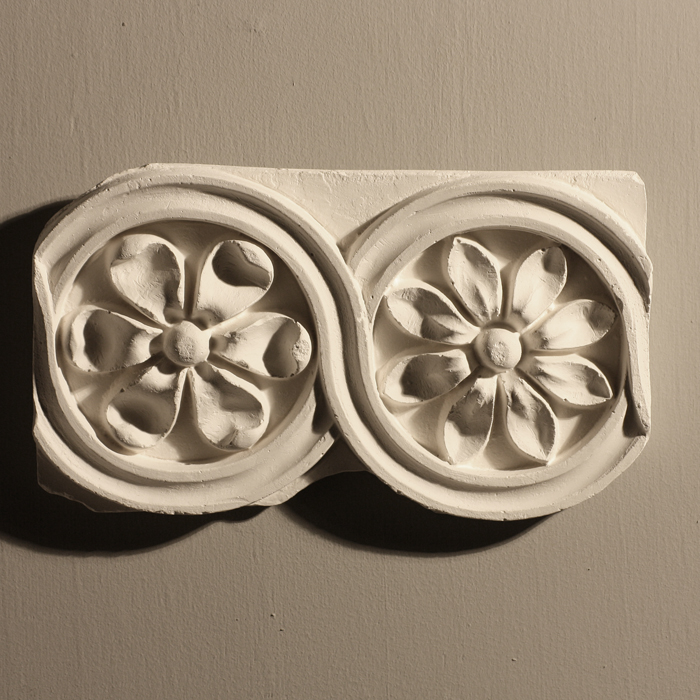The image depicts an intricately molded sculpture resembling a horizontal figure-eight or infinity symbol, with each loop containing a detailed floral design. The sculpture appears to be made of a white or off-white clay or ceramic material. The left loop features a flower with six broad petals and a prominent pistil at the center, while the right loop displays a flower with eight narrower petals and a distinct pistil. The entire piece is presented against a light gray to beige background that contrasts subtly with the object's creamy hue. The lighting, coming from the top right, casts a gentle shadow towards the left and down, adding depth and dimension to the sculpture. This elegant piece captures the delicate nature of floral forms within a structured, interconnected design.